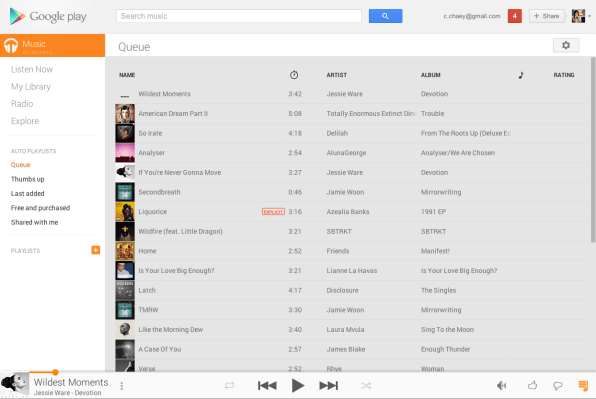**Screenshot of a Google Play Music Playlist**

The image is a detailed screenshot of a Google Play Music playlist, oriented in landscape mode. At the top of the screen, a gray bar stretches across the width, featuring the "Google Play" logo on the left side with its signature multicolor triangle arrow. Adjacent to the logo is a search bar, containing the placeholder text "Search music". To the right of the search bar is a blue button with a magnifying glass icon, intended to initiate a search. Further right, there is some text and a tiny user profile photo, though the text is too unclear to read.

On the left side of the screen, a white column is topped with an orange header bar labeled "Music". This column contains several menu options including "Listen Now", "My Library", "Radio", and "Explore", followed by "Auto Playlist" categories like "Queue", "Thumbs Up", "Last Added", "Free and Purchased", and "Shared with Me". The "Queue" option is highlighted in orange, indicating that it is currently selected. Below these options is a section labeled "Playlist" with a plus sign inside an orange square, presumably for adding new playlists.

The main area of the screen, which has a gray background, displays detailed information about the playlist. This includes columns for the song name, length, artist, album, and rating. The playlist listed features 14 songs. The second song displayed, "American Dream", bears a square thumbnail of its album cover. The first song in the list is "Wildest Moments" by Jessie Ware from the album "Devotion", with a duration of approximately 3 minutes and 42 seconds.

At the very bottom of the screen, there is a control bar indicating that "Wildest Moments" is currently playing. This bar includes play, rewind, and fast-forward buttons, among other icons that are not clearly identified.